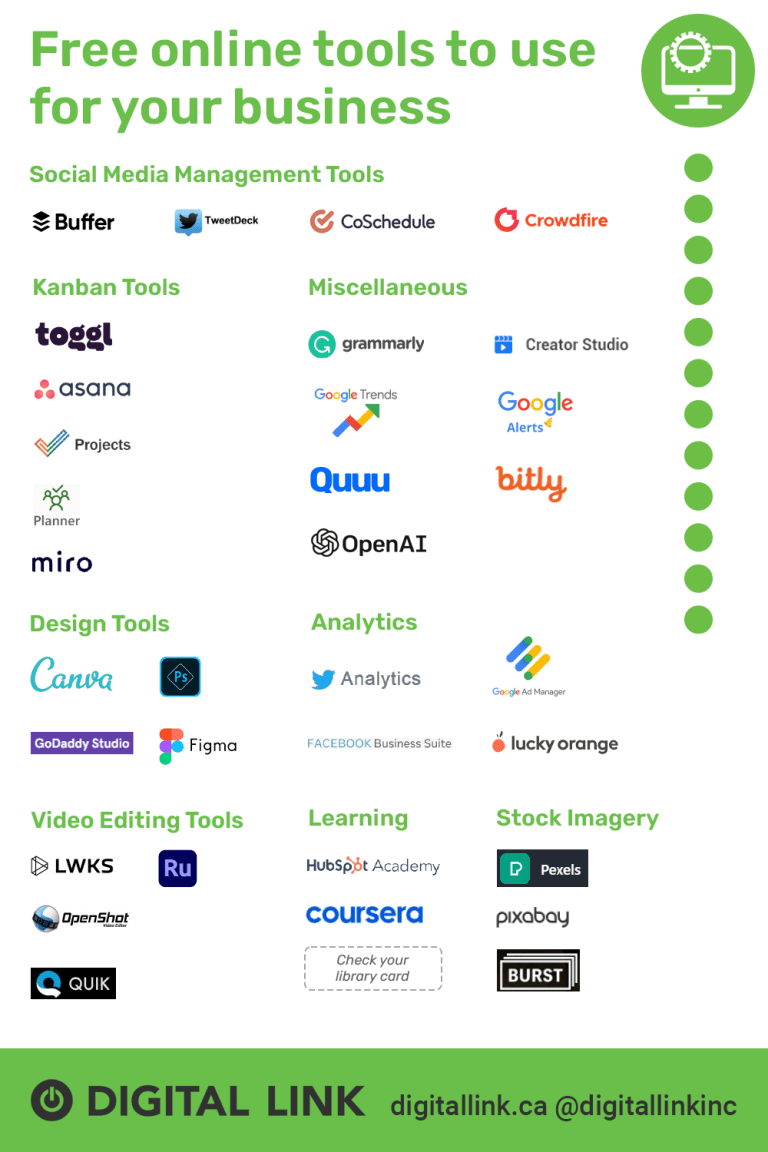**Advertisement Screenshot: Comprehensive Business Tools**

This vertical advertisement features a clean white background with clearly structured content. At the very top, in bold green text, it announces "Free Online Tools to Use for Your Business." Directly below in a slightly smaller font, the heading "Social Media Management Tools" is displayed.

To the right, there is a prominent green circle containing a white icon of a desktop monitor adorned with a gear symbol, indicating a focus on tools for management and efficiency. Beneath this icon, there is a vertical series of 12 green dots, adding a visual flow to the ad.

On the left-hand side, a variety of company logos and tool names are neatly categorized under different headings:

1. **Social Media Management Tools**:
    - Buffer
    - TweetDeck
    - CoSchedule
    - Crowdfire

2. **Kanban Tools**:
    - Toggl
    - Check
    - Projects and Planner
    - Miro

3. **Design Tools**:
    - Canva
    - Photoshop
    - GoDaddy Studio
    - Figma

4. **Video Editing Tools**:
    - LWKS
    - OpenShot
    - Quik

5. **Miscellaneous**:
    - Grammarly
    - Creator Studio
    - Google Trends
    - Google Alerts
    - Q
    - Bitly
    - OpenAI

6. **Analytics**:
    - Twitter Analytics
    - Facebook Business Suite
    - Google Ad Manager
    - Lucky Orange

7. **Learning**:
    - HubSpot Academy
    - Coursera

8. **Stock Imagery**:
    - Pexels
    - Pixabay
    - Burst

This advertisement efficiently compiles a diverse array of essential tools and resources for businesses, highlighting options for social media management, project planning, design, video editing, assorted utilities, analytics, educational opportunities, and stock image resources.